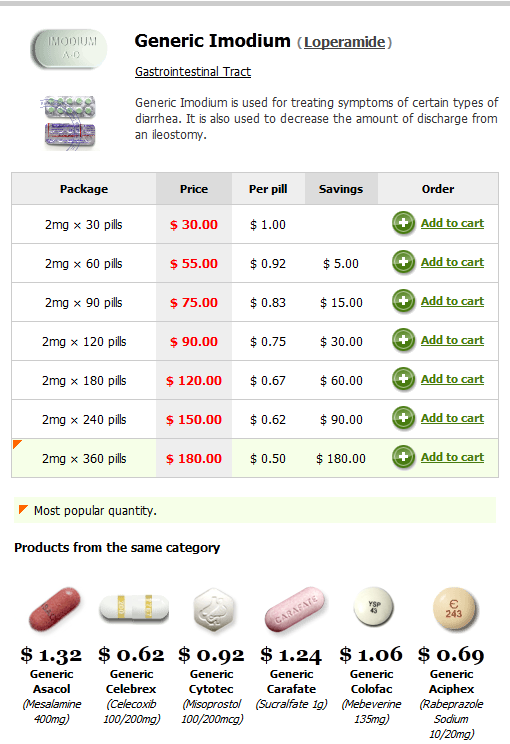**Image Description: Detailed Pill Comparison Guide for Imodium (Loperamide)**

This image is a comprehensive screenshot depicting a comparison guide for the medication Imodium, whose generic name is loperamide. At the focal center of the image, the text "Generic Imodium (Loperamide)" is prominently displayed in parentheses. 

To the upper left corner of this central text, there is an image of a branded Imodium pill. Directly beneath this image, the term "Gastrointestinal Tract" is written in all capitals. Following this, a brief description provides information about Imodium: "Generic Imodium is used for treating symptoms of certain types of diarrhea. It is also used to decrease the amount of discharge from an elastomy."

Moving further down, to the left of the text, the image showcases two separate Imodium pills or packages still enclosed in their blister packs. Below these blister packs, a detailed price comparison chart is displayed. This chart outlines the cost per package for varying quantities, starting from a 2 mg dose for 30 pills and extending up to 360 pills. The chart also includes information such as the price per pill, total savings, and order options.

At the very bottom of the image, a section lists similar medications within the same category, along with their respective prices, offering a complete overview for comparison purposes.